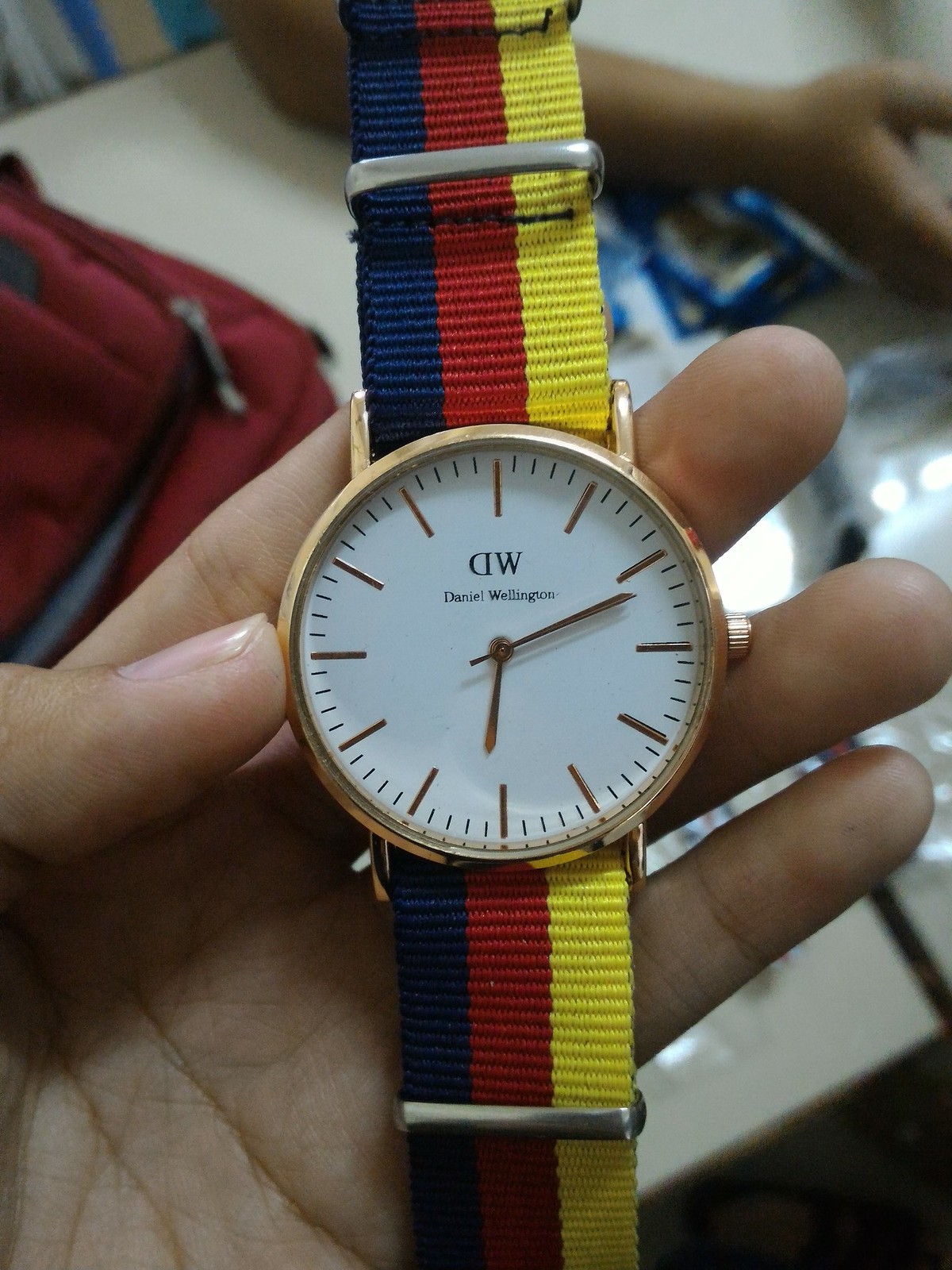A close-up image of a polished wristwatch is displayed. The watch features a sleek white face adorned with elegant gold accents. Instead of traditional numerals, simple gold lines mark the hours, contributing to its minimalist and sophisticated design. The brand "Daniel Wellington" is prominently inscribed on the face, identified by the iconic "DW" logo. The watch is positioned on the wrist of a fair-skinned individual.